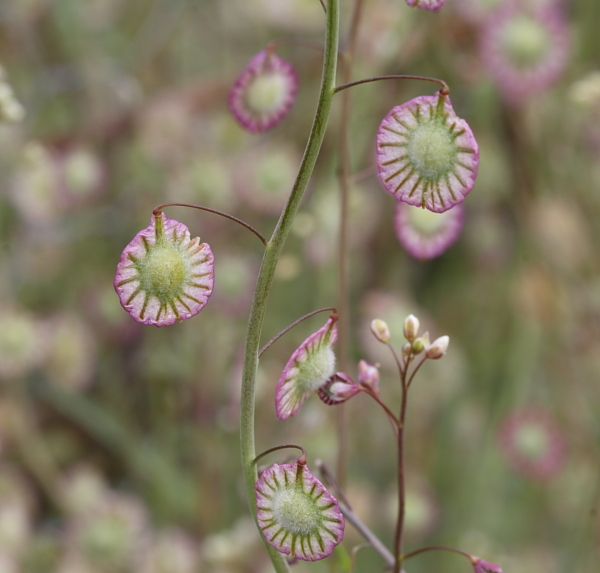In this square-shaped photograph, a close-up captures two prominent plants in the foreground, set against a blurry backdrop of similar foliage. The main plant features a long green stem with thin, reddish-brown branches extending at wide intervals. Each branch culminates in a round, coin-sized flower, amounting to about four to seven per plant. These flowers are striking, with a green center resembling a sun, from which vein-like lines radiate outward to a purple border. The intricate pattern makes each flower appear as if it has a green and brown star at its core, encircled by a vivid purple edge. Additionally, the plant on the right displays predominantly white, unopened buds at its tip, while the left plant showcases round, flat seed pods that alternate along its stem. These seed pods have a light green bulging center and are encased in a translucent, paper-thin disc with purple edges, mirroring the flower’s intricate vein-like spikes extending from the center to the perimeter.